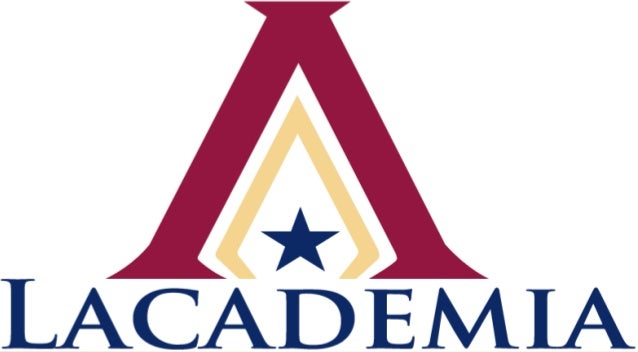The logo features a central, prominently large letter "A" in a dark red hue with sharp corners. This "A" lacks the typical horizontal bar, and in its place, there's a pale gold, triangular outline. Within this outline rests a navy blue, five-pointed star, situated above the word "Lacademia." The text "Lacademia" appears in a serif font and is also navy blue, slightly offset to the right of the central shapes. The entire logo, comprising the red "A," the gold outline, the blue star, and the navy blue text, is set against a pure white background.